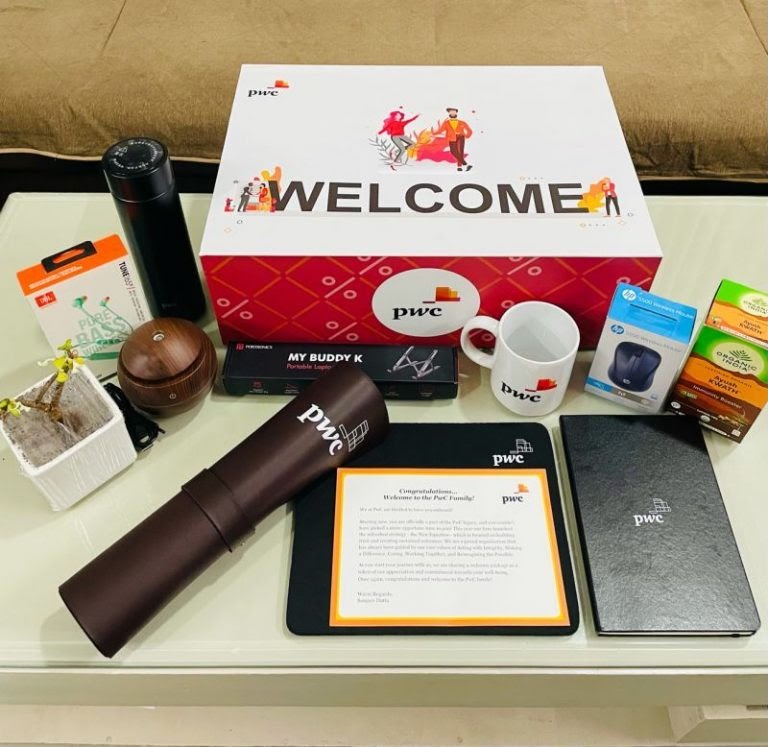The photograph is a full-color, staged indoor scene taken with natural light, featuring a square format without any borders or distinctive background elements. Central to the composition is a white table, possibly covered with a glass top, on which various items are meticulously arranged. Dominating the top center of the table is a large 'Welcome' box, reminiscent of a donut box, adorned with artistic images of six cartoon-style people (three men and three women). The box has a striking design with a white top and red sides displaying a crosshatch graphic.

Several items on the table bear the PWC logo, including a white coffee cup, a leather notebook, and some type of tube-shaped object. Additional items include a blue box, a green and brown box, and what appears to be a small plant in a square pot. There's a brown couch in the background, partially visible with just the cushion part showing. Among the diverse assortment of gifts are a Moleskine notebook, a mouse pad, a pepper grinder, a My Buddy K portable laptop stand, a small HP portable mouse, organic India green tea, headphones, a wooden orb-like object with a power button, and a black cylinder which might be a water bottle or power bank. A pot with yellow flowers adds a dash of color and a touch of nature to the setting.